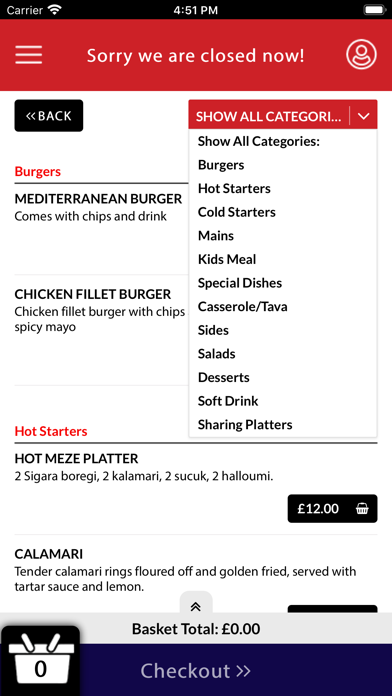The image displays a food delivery app interface. At the top, the status bar shows the carrier, Wi-Fi symbol, the time (4:51 p.m.), and the battery indicator. A prominent red banner with white text reads, "Sorry, we are closed now." Below this, there's an outline of the top of a person's head within a white circle, a black back button, and a drop-down list labeled "Show all categories" in bold text.

The categories listed include:
- Burgers
- Hot Starters
- Cold Starters
- Mains
- Kids Meal
- Special Dishes
- Casseroles
- Hashtava
- Sides
- Salads
- Desserts
- Soft Drink
- Sharing Platters

The "Burgers" category, highlighted in red, details a Mediterranean Burger that comes with chips and a drink, and a Chicken Filet Burger with chips and spicy mayo. The "Hot Starters" section lists a "Hot Me's Platter" which includes two portions each of Tigeria Borgie, Calamari, Saku, and Halloween for £12. Another option is Calamari, described as tender calamari rings floured and golden fried, served with tartar sauce and lemon.

At the bottom of the screen, it states "Basket Total: £0" next to a cart icon with the number zero, and a purple "Checkout" button.